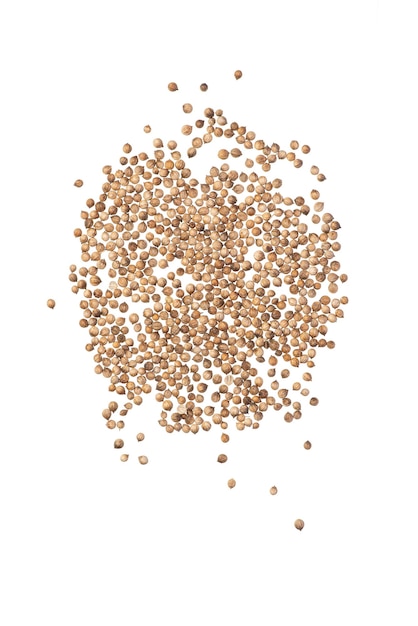The color photograph, taken indoors under bright lighting, showcases a close-up of a dense, rounded cluster of tan, light brown, and dark brown nuts. The nuts, displayed against a stark white background, are likely shelled walnuts or almonds, though their exact type is unclear. Arranged in a somewhat circular pattern, the collection consists of three to four hundred nuts, densely packed in the center and gradually becoming sparser towards the edges. The nuts lie flat in a single layer, with a few scattered randomly outside the main cluster. The meticulous arrangement and bright lighting suggest the purpose of the image is to advertise or sell the nuts, emphasizing their uniformity and color variations. With no other objects or distractions in the frame, the clear focus is on the nuts themselves, making for a visually striking and detailed display.